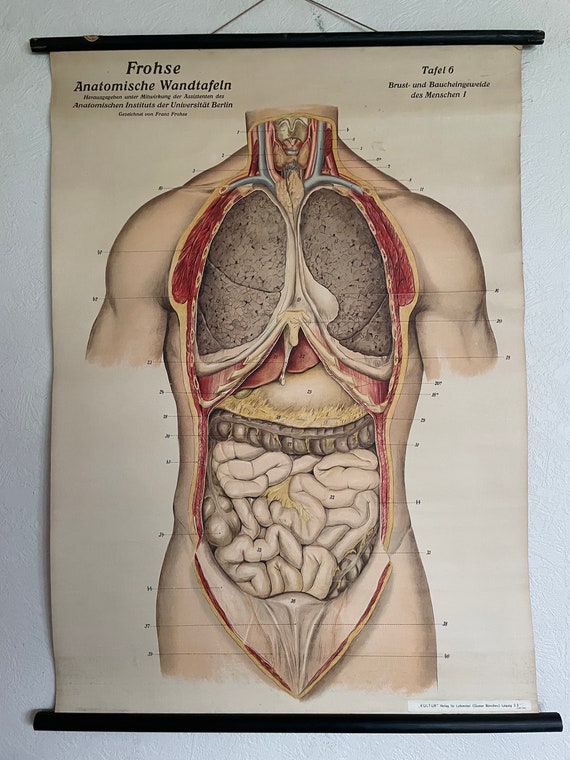The image depicts an old, hanging anatomical diagram of the human body, likely from the 1950s, displayed against a light-colored wall, possibly white or grayish. The poster is mounted on a black horizontal strip at both the top and bottom, and is suspended by a small rope or strings attached to a nail in the wall. The diagram is detailed, showing the torso with the skin peeled back to reveal internal organs. Visible are the lungs, heart, liver, pancreas, stomach, intestines (including the colon and small intestine), neck with arteries and veins, pelvis region, shoulders, and the upper parts of the arms and legs. Numbers are printed around the diagram, indicating different areas inside the body, but there is no accompanying key. The text and numbers on the poster are in black and appear to be written in German, suggesting it might be from a German institute.